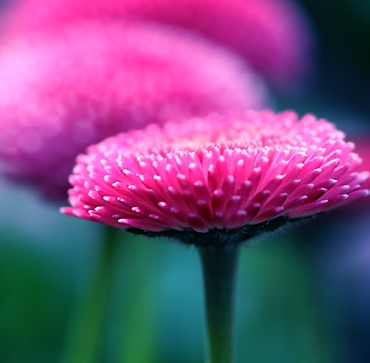This image showcases a vivid, zoomed-in close-up of a pink flower dominating the bottom half of the frame. The flower is adorned with numerous pink petals, making it appear almost monochromatic, with the exception of its dark green stem that has a fuzzy base. Surrounding the main flower, the background is blurred, enhancing the focus on the primary bloom. In this blurred background, there are glimpses of at least two other similar pink flowers, which might be actual flowers or their reflections. The backdrop displays a gradient of colors, transitioning from dark green at the bottom left to dark blue at the bottom right, with a hint of black in the top right corner. The overall scene, whether natural, printed, or painted, exudes a striking vividness and is bathed in a spectrum of hues that accentuate the stunning pink flower in the forefront.